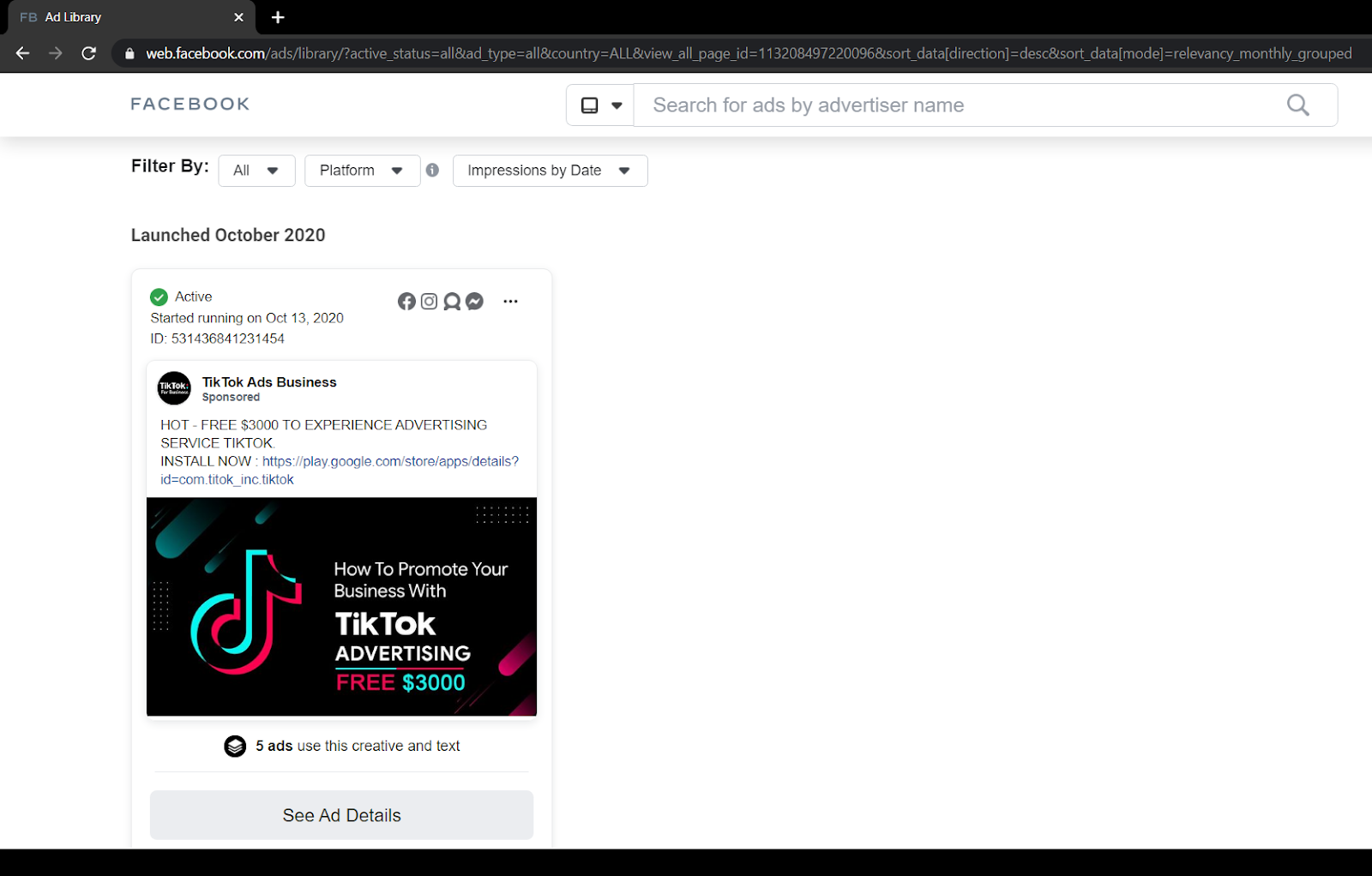In this image, we observe a webpage with a visible browser tab that displays an active link. The URL featured is part of the description for a video hosted on YouTube, and the specific link shown is "https://www.youtube.com.ac". The web page appears to focus on details relevant to the video content, indicated by the contextual placement of the URL within the description section.